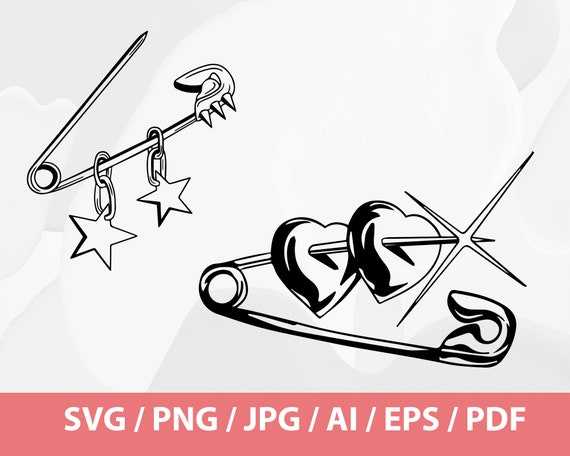The illustration features two black and white vector-style safety pins set against a square canvas with a coral-pink horizontal strip at the bottom. The safety pin in the upper left corner is open, with three small, triangular spikes on the clasp end. Dangling from this pin are two chain links, each adorned with a star charm. Positioned in the bottom right corner, the other safety pin is also open and features two hearts impaled on its shaft. A sparkling effect is illustrated at the pin's point. Beneath the pins, the coral-pink strip displays white text listing various vector file formats: SVG, PNG, JPG, AI, EPS, and PDF. The overall style of the artwork is clean and illustrative.